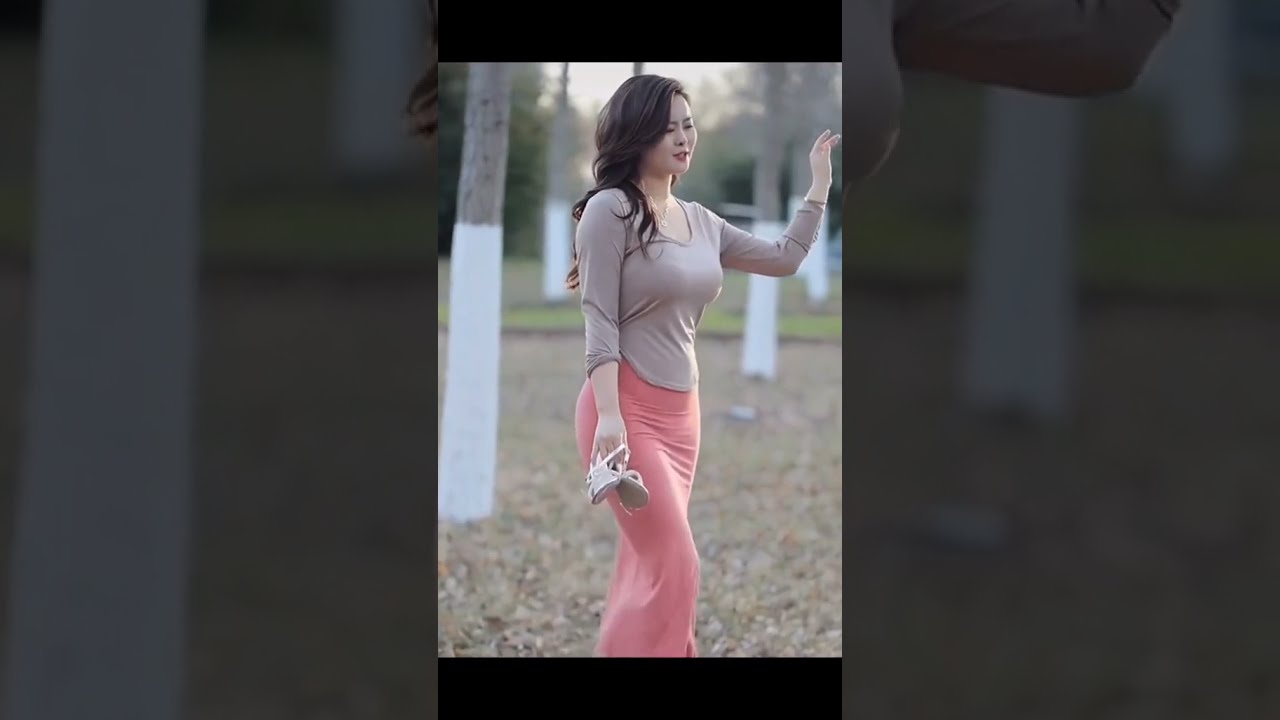This photograph features an Asian woman with long, wavy black hair and wearing makeup, standing outdoors amidst some trees. She is donned in a beige long-sleeve shirt and a flowing pink skirt or pants. The ground beneath her appears to be covered in what could be dirt, leaves, or mulch, rather than grass. The trees in the background have their trunks painted white up to three or four feet, with the bark visible above the white coating. 

The woman, positioned centrally in the image, is looking slightly downwards and not at the camera, possibly giving the impression of waving or reaching for something with her left hand raised and bent at the elbow. Her right hand holds a pair of sandals. The image showcases various colors such as black, white, gray, brown, off-white, pink, green, and hints of yellow, red, and tan. The ambient light suggests it’s daytime, and the outdoor setting is further emphasized by a glimpse of the sky and blurry greenery in the background. The photograph’s edges are darkened, focusing attention on the subject in the center, as if it were possibly a screenshot from a mobile app like TikTok or Instagram live stream.